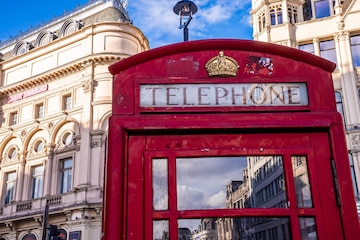The image showcases an old-fashioned red English telephone booth set against a vibrant city backdrop. Prominently featured at the top of the booth is a gold crown above the word "TELEPHONE" inscribed on a white background. The booth’s glass windows are reflective, capturing the essence of the surrounding cityscape, including hints of cars and possibly a double-decker bus, suggesting the scene is set in London. Flanking the booth are grand, white, multi-story buildings adorned with arched windows. The left building appears triangular due to the angle of the shot, enhancing the architectural charm. Above, a clear blue sky with minimal clouds stretches across the scene, highlighting the striking contrast between the antique charm of the telephone booth and the expansive urban environment.